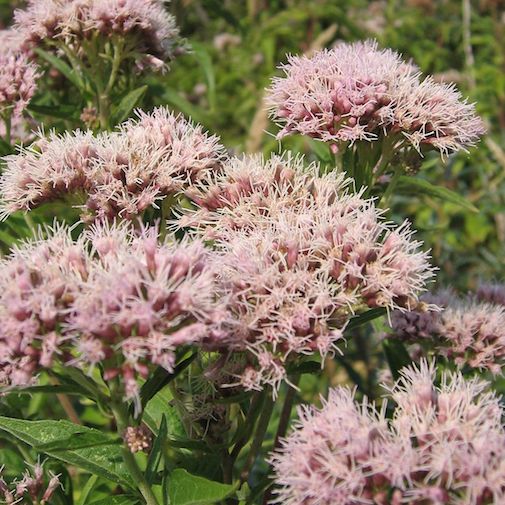This close-up photograph captures an array of pink, spindly, and densely clustered flowering plants amid a backdrop of green leaves and stems. The scene, taken during the day, showcases approximately seven to fifteen flower buds in sharp relief. The flowers, resembling thistles with a lavender-pink hue, appear waxy and are emerging from a green base. No text, insects, or animals are present in the image, and the green background is somewhat blurred. While the photograph isn't professional, it effectively highlights the natural beauty and intricate details of the plant life.